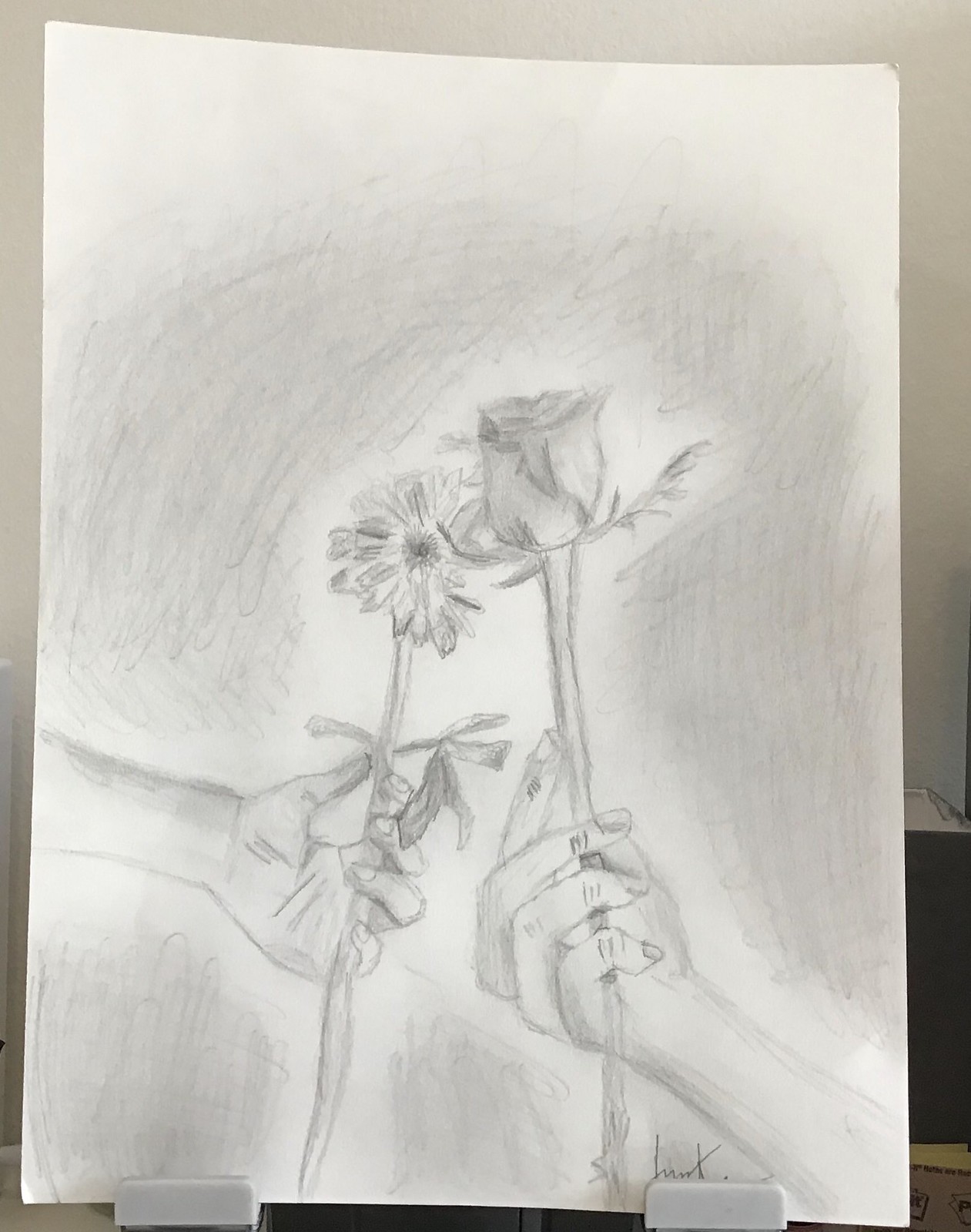The image depicts a detailed sketch on a piece of paper. The focal point of the drawing is a hand extending from the right-hand side, with fingers curled delicately around the stem of a partially bloomed rose. The petals of the rose are closed, showing signs of an upcoming full bloom. Leaves are visible, protruding from the bottom of the flower bulb, adding to the intricate detailing of the sketch. There's a notable black dot in the center of the flower. The background features subtle shadowing, adding depth to the illustration. Previously, there were scratchy marks around the bottom left and throughout the background, which have since been mostly erased. The artist's signature is located in the bottom right corner, marking their completion of this elegant and detailed botanical drawing.